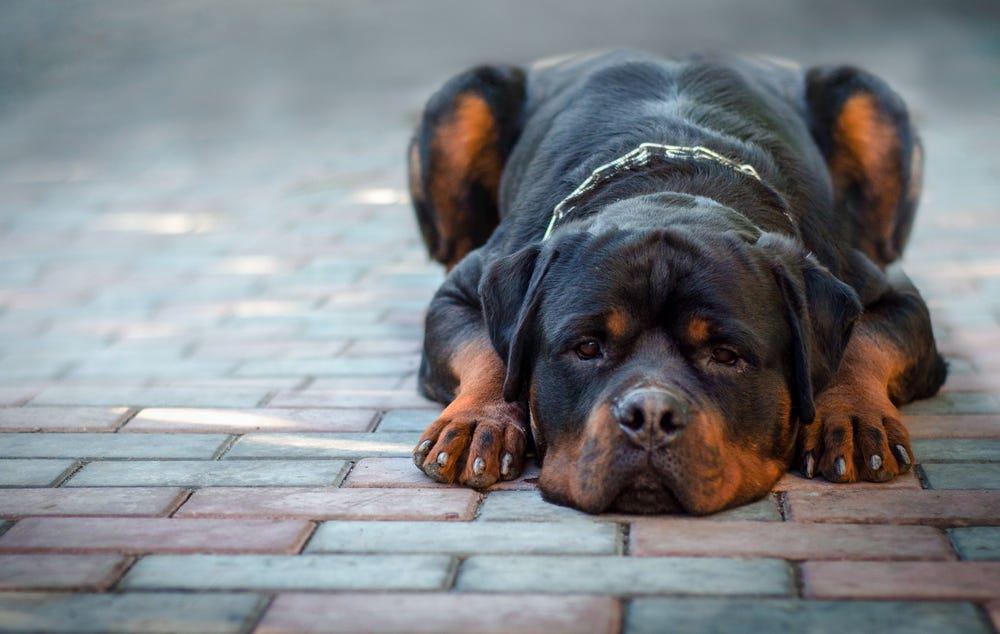In the image, a Rottweiler dog lies on a brick paved pathway, which comprises varying colors of red, gray, and orange. The dog is positioned towards the center right of the frame, exhibiting a slightly melancholic expression as it looks directly into the camera. The Rottweiler, which appears to be an older dog, has a mostly black coat accented with light brown markings, including distinctive spots above its eyes and on its forelegs and muzzle. It wears a metal chain collar around its neck. The dog is lying submissively with its front paws flat on the ground and its hind legs slightly raised. The setting is illuminated by rays of light shining on the brick floor, highlighting the dog's recently trimmed nails. The atmosphere suggests the dog might be feeling contemplative, possibly because it is not being allowed to play or is in some form of trouble.